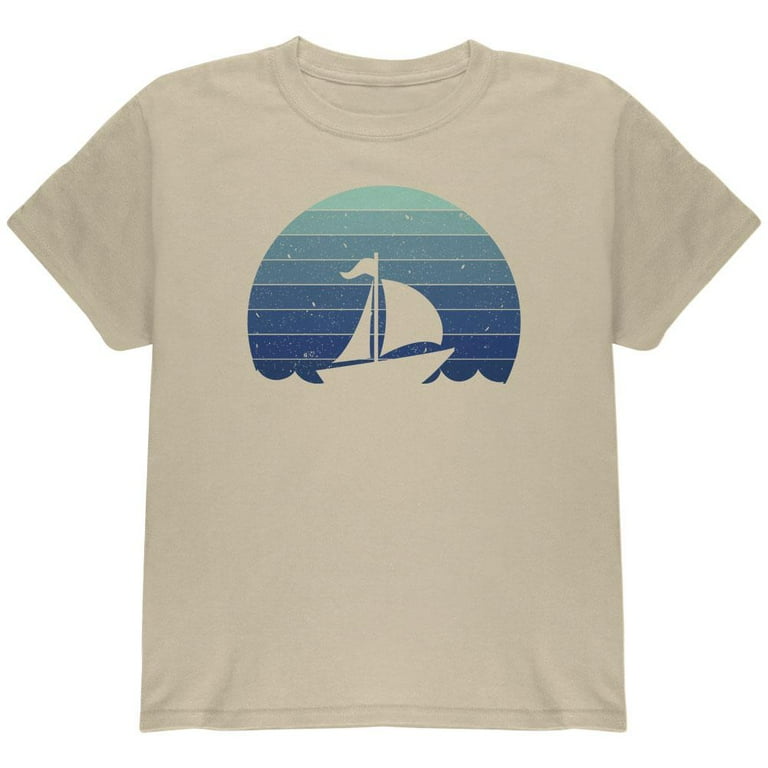The image displays a beige short-sleeved t-shirt with a crew neck, neatly laid out against a white background. The shirt, featuring stitching across the bottom hem, stands out with a central design. This design is a semicircle filled with horizontal gradient stripes that transition from light turquoise blue at the top to indigo at the bottom, giving the appearance of ocean waves where the semicircle is cropped. Within this gradient, a white sailboat with a visible flag seems to sail across the waves, adding a serene nautical touch to the otherwise plain t-shirt.